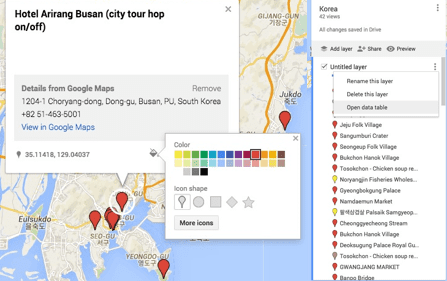A detailed map of South Korea is pictured, featuring multiple pins indicating various locations. One prominent pin has a large white box, similar to a speech bubble, which reads, "Hotel Arirang Busan City Tour Hop on off." Below this, a smaller gray box displays additional details from Google Maps with some numbers and letters, along with the text "South Korea." A visible option allows users to view this map in Google Maps. The map interface includes a color adjustment tool, with a box open showing pins being changed to red. On the right side, a comprehensive list of options is visible, including "Korea," "rename this layer," "delete this layer," and "open data table." The list of pins primarily shows red indicators, with the exceptions of two yellow pins and one light brown pin. There’s also a highlighted blue or black square around the red color option, indicating that this is the current selection for most of the pins on the map.